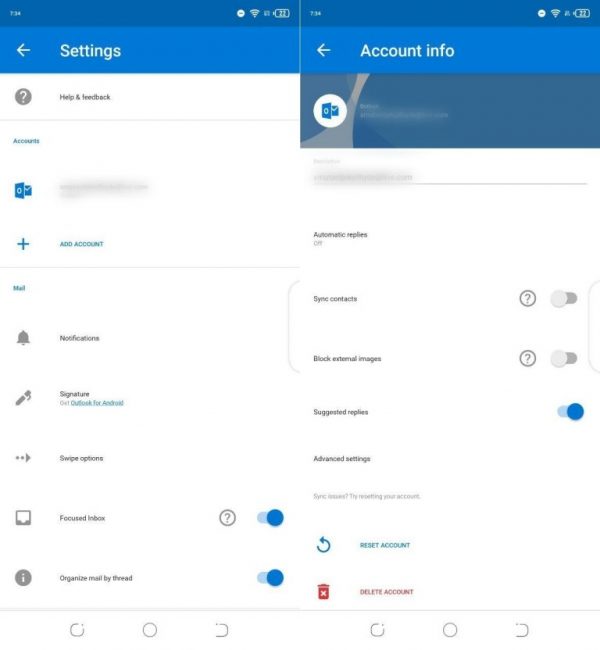The image consists of two side-by-side screenshots from a mobile device's settings pages, both topped with blue navigation bars. The left screenshot is labeled "Settings," and the right one is labeled "Account Info." 

On the left side, several sections are displayed, each accompanied by an icon. At the top, "Help & Feedback" is signified by a question mark icon, followed by "Accounts" below it. One account entry is blurred out, and there's an option with a plus sign labeled "Add Account." This section is designated as "Mail" and includes various settings such as "Notifications," "Signature," "Swipe Options," "Focused Inbox," and "Organize Mail by Thread."

The right screenshot focuses on account-specific settings under "Account Info." It features a blurred email address next to a mail icon and a blurred top bar. Directly beneath, it states "Automatic Replies Off." Further options include a toggle for "Sync Contacts," which is on the right, and "Block External Images," with the toggle switched off. The "Suggest Replies" toggle is active and highlighted in blue. The section concludes with "Advanced Settings," offering actions such as "Reset Account," identified by a refresh icon, and "Delete Account," marked with a red trash can icon.